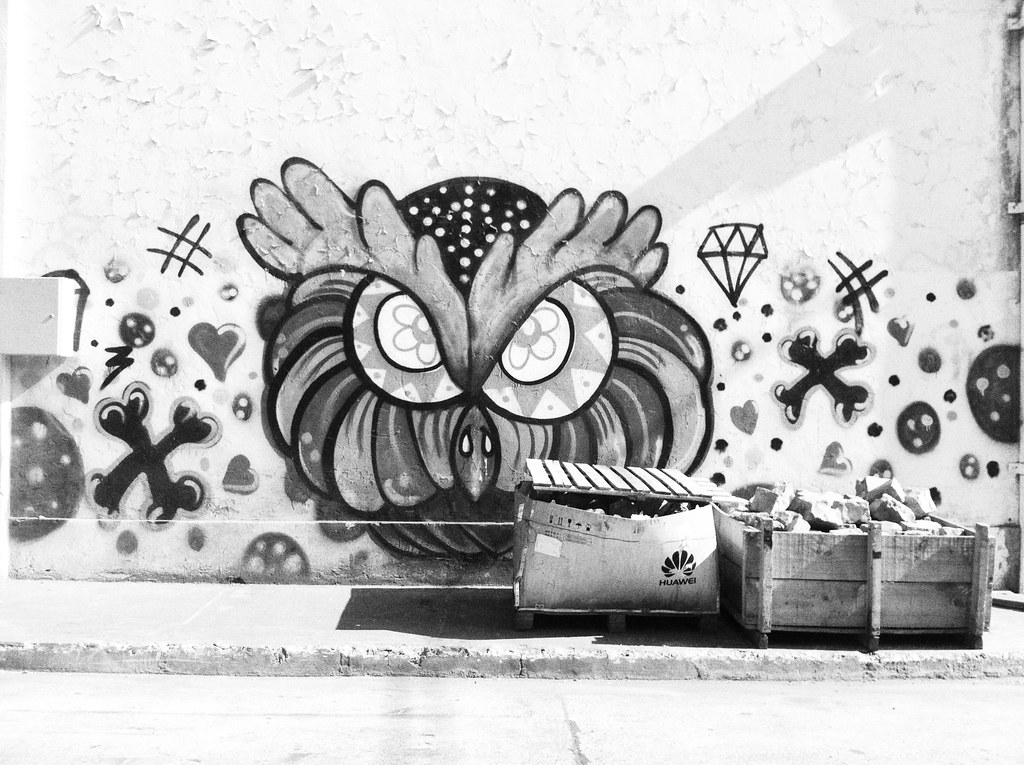The black and white image features a textured, possibly peeling, light-colored wall covered in detailed graffiti art. Dominating the center is an intricately painted owl with an angry expression, characterized by large eyes with floral patterns in the irises, puffy feathers, and a beak prominently displayed. Above the owl's head, there's a speckled area adding to the depth of the design. To the left and right of the owl, there are crossed bones, with the right-side bones positioned higher and appearing smaller. Additionally, a stylized diamond is situated near the right-side bones. Surrounding the central owl are a mix of filled-in hearts and circular shapes, along with some hashtags, adding to the graffiti's complexity. In the foreground, on the sidewalk, there are several boxes, one labeled "Huawei," seemingly filled with rough rocks.